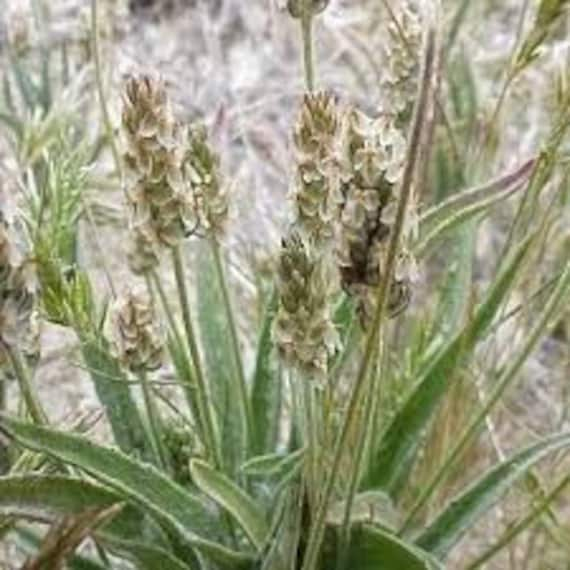This vertical rectangular photo captures a plant with white, cylindrical clusters of small flowers, framed against a backdrop that resembles ice-covered vegetation. The image's clarity, while not the sharpest, allows for detailed observation of the plant's features. Central to the composition are green stems, varying in thickness from slim to roughly finger-width, with some stems curving backward. These stems support the flower clusters, which consist of numerous small, pale gray to white petals. The plant features about five or six of these flower-stalks, giving a somewhat cylindrical appearance overall. Surrounding the plant are long, green grassy leaves, contrasting with the background of dead, beige-colored grass, adding to the sense of an outdoor setting possibly in a field or trail area. The colors in the image are muted, contributing to its somewhat dull appearance.